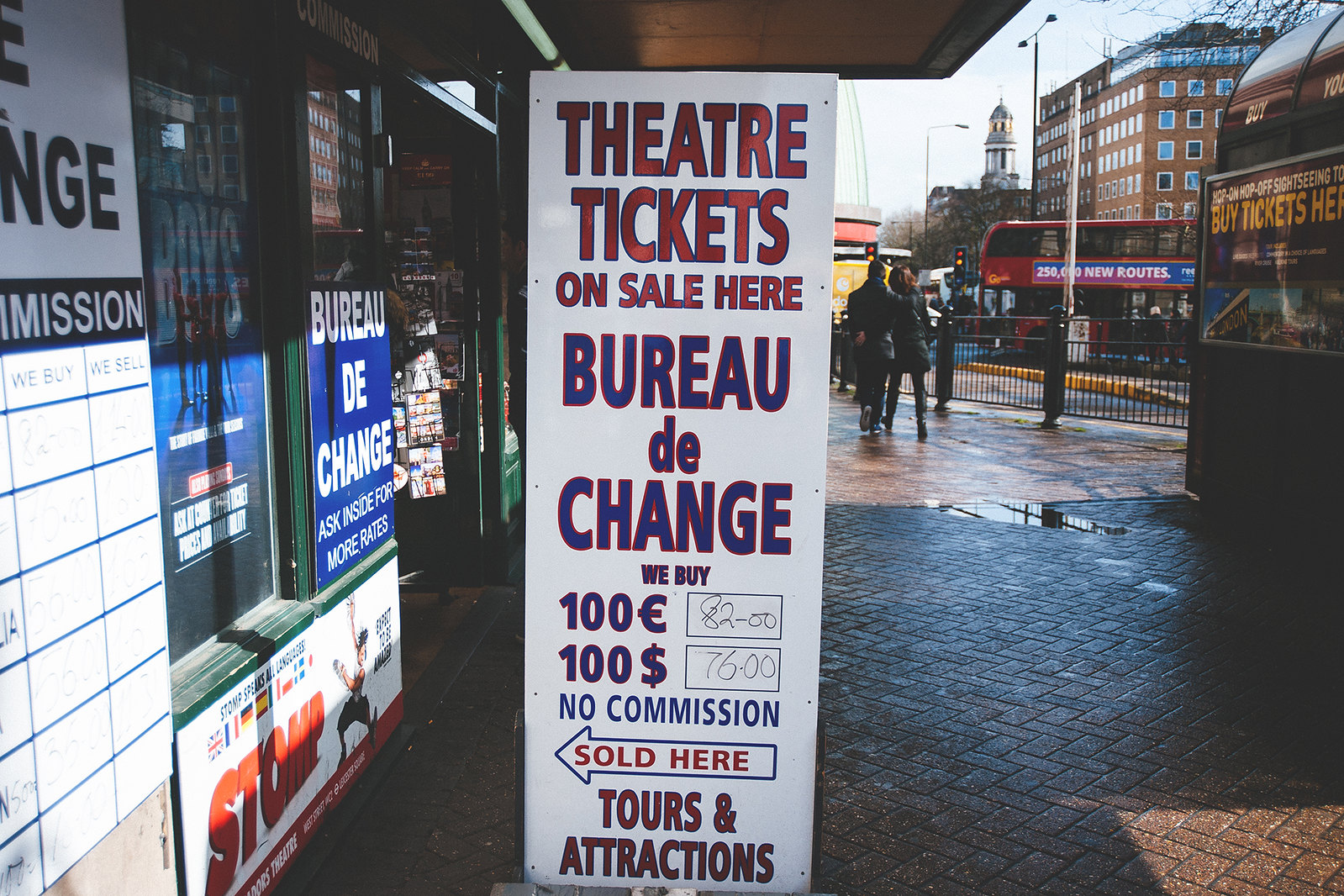The image depicts a lively urban street scene with a cobblestone walkway and an older apartment building in the distance. A red double-decker bus is parked by the street, suggesting the scene might be in London. The sidewalk features black grating or fencing, adding to the bustling city atmosphere. Centrally, a prominent white sign next to a storefront captures attention. The sign, in bold red letters, advertises "Theater Tickets on Sale Here," and in blue letters below, it reads "Bureau de Change." It details currency exchange rates, stating "We buy 100 Euros" and "We buy $100," with noted rates of 82 pounds for euros and 76 pounds for dollars. The sign also mentions "No Commission" and includes an arrow pointing left, directing passersby to shops nearby for tours and attractions.